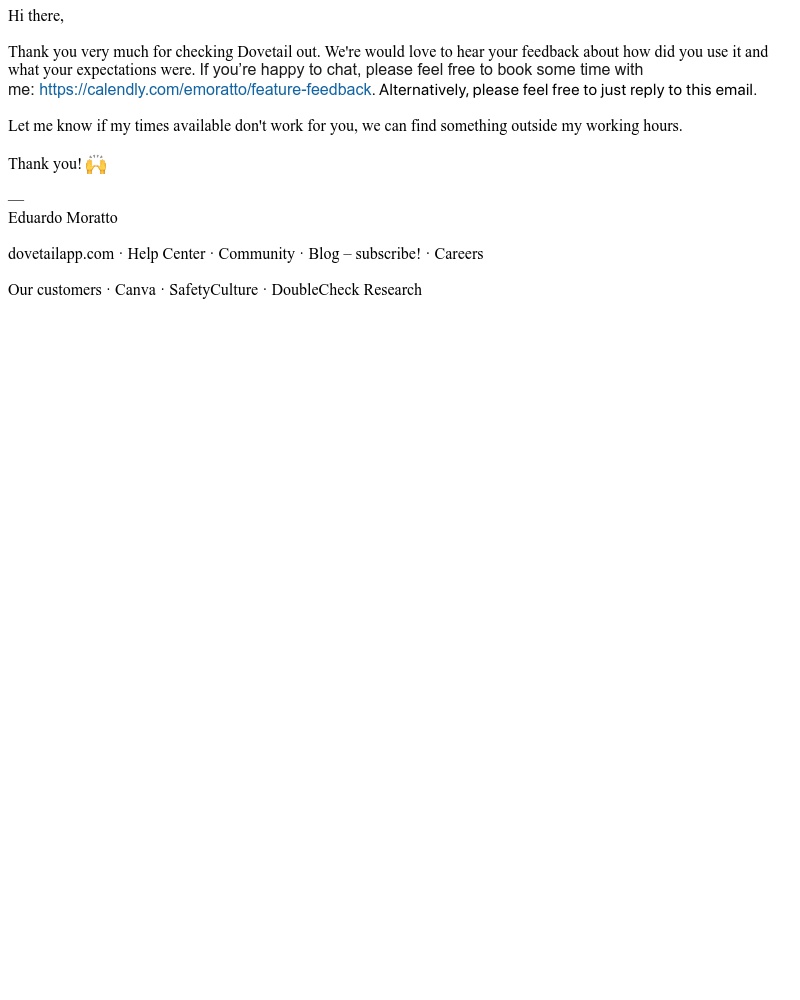The image features a predominantly white background. At the top section, there is a blank white area. Below this, in black text, it reads:

"Hi there, thank you very much for checking Dovetail out. We would love to hear your feedback about how you used it and what your expectations were. If you're happy to chat, please feel free to book some time with me."

Following this message, there is a blue hyperlink: "https://kallenlee.com/emiratic/feature-feedback". The text continues:

"Alternatively, please feel free to just reply to this email. Let me know if my available times don't work for you; we can find something outside of working hours. Thank you."

Underneath, there are two hands up in the air emoticons. Beneath a horizontal line, it reads:

"Eduardo Morado,
Dovetailapp.com, Help Center, Community, Blog, Subscribe, Careers, Our Customers, Canva, Safety Culture, and Double Check Research."